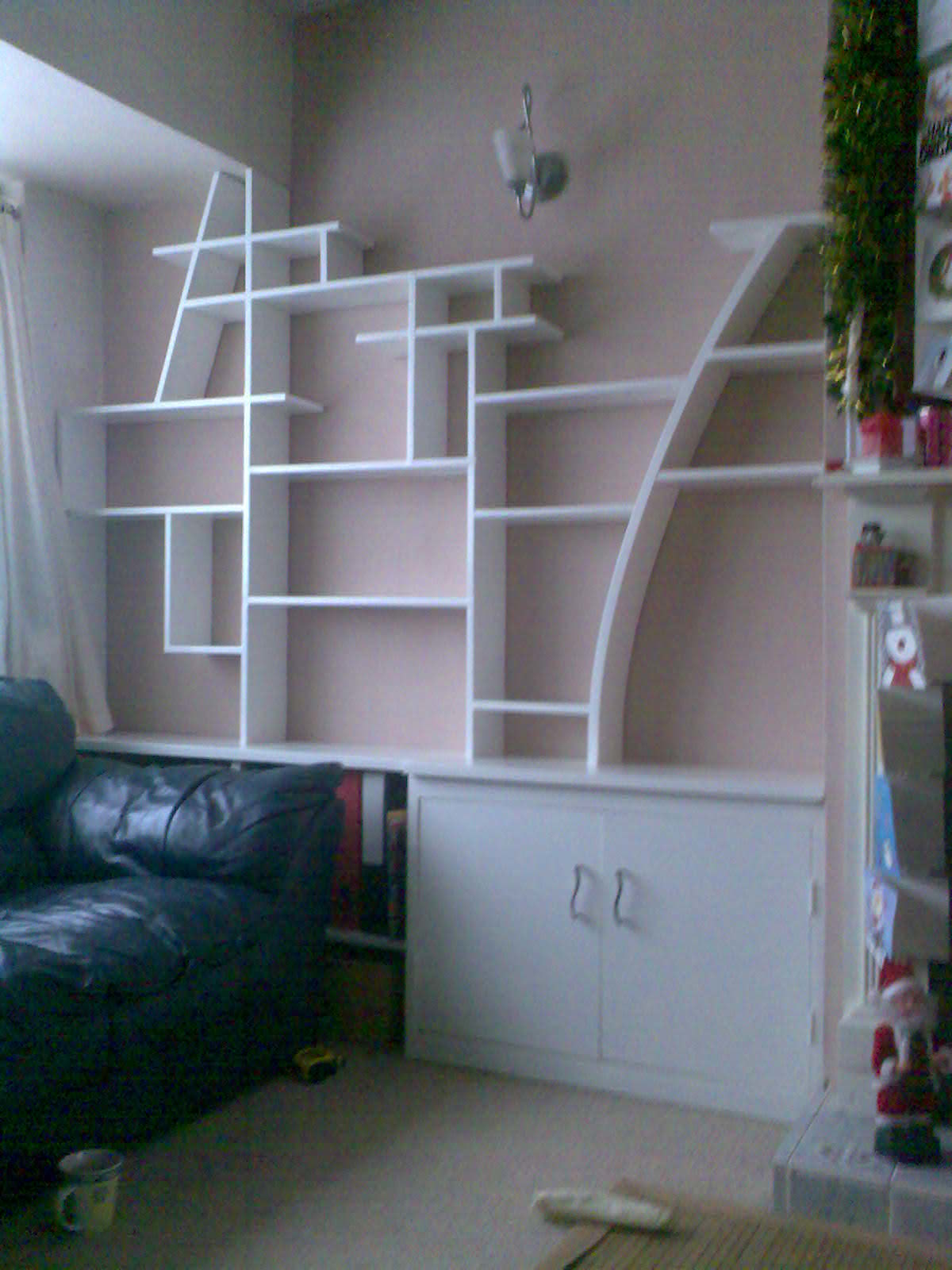This grainy color photo captures an eclectic living room scene with a pinkish-beige wall adorned with unusual built-in shelving. The eye-catching shelves are a mix of rectangular and arching shapes, resembling the top of a rowboat or a canoe, and are designed in a seemingly random pattern that includes intersecting white lines. Below the shelves are white double-door cabinets and open bookshelves, providing additional storage space. A silver and glass sconce is mounted above the shelves, illuminating the arrangement.

In the right-hand side of the image, a fireplace mantle appears, partially decorated with Christmas items such as a small Santa Claus figure, decorative garlands, red candles, and potentially a faux topiary Christmas tree-shaped ornament. The bottom right corner also displays more festive decor.

On the left side of the room, a well-worn black or dark leather couch sits beneath a window with a white curtain, flanked by a coffee cup on the ground. The room seems quite empty and possibly slightly disordered, contributing to the overall impression of a space not currently in active use. The presence of wall-to-wall carpet and a dog bone on the floor adds to this impression, giving it a somewhat deserted or transitional feel.